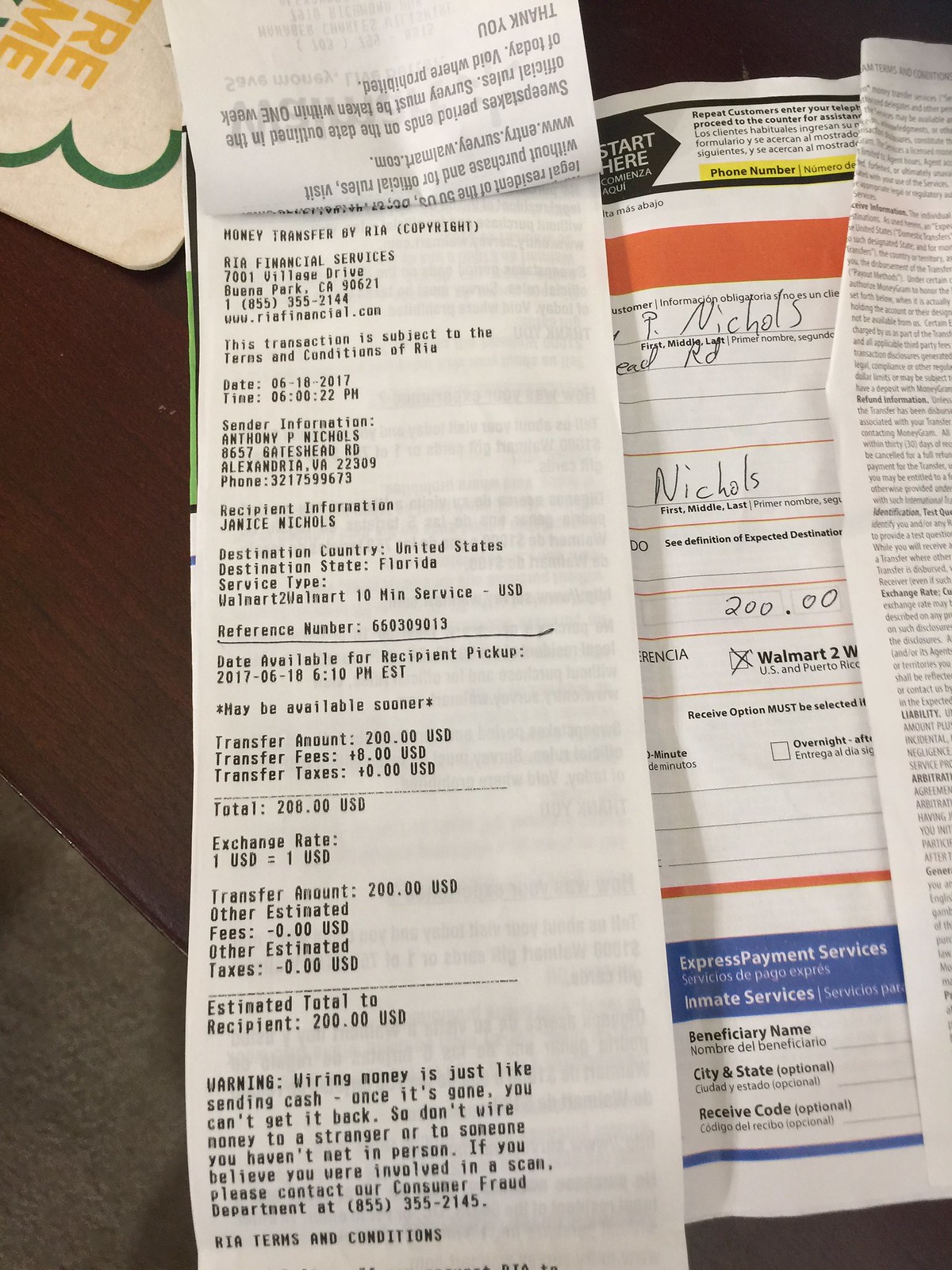A detailed caption for the image could be:

"This is an image of a purchase receipt detailing a wire transfer of funds. The receipt, printed in black lettering, is titled 'Money Transfer' at the top and was issued by A-One Financial Services, whose address is provided on the document. The sender information lists Anthony Nichols along with his address, while the recipient is noted as Janice Nichols. The transfer amount specified is $200 USD. In the background of the image, a table is visible, and to the right, other paperwork related to the wire transfer is scattered, providing additional context to the transaction."